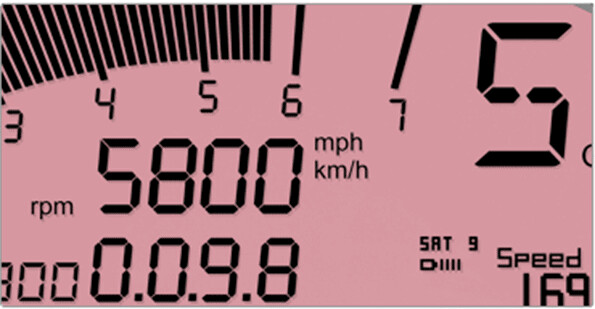This image features what appears to be a digital speedometer, though it’s unclear if it is real or computer-generated. The backdrop is a vivid pink, giving the scene a striking visual effect. The display is somewhat truncated, revealing partial yet significant data. Centered on the screen is the label "RPM" followed by the number 5800, indicating revolutions per minute. Adjacent to this, the terms "MPH" and "KM/H" denote measurements in miles per hour and kilometers per hour, respectively. Below, a series of numbers appear, though they are incompletely visible due to the image’s cropped nature. To the right, the word "Saturday" and the numeral "9" likely reference a date. The speed reading is partially obscured but shows "169," suggesting a high velocity. Above, a large numerical "5" is visible but also partially cut off. There are black vertical bars in the top left corner of the display, indicating some form of measurement. The incomplete and fragmented nature of the image adds a layer of ambiguity as to whether the data presented is real or generated by software.